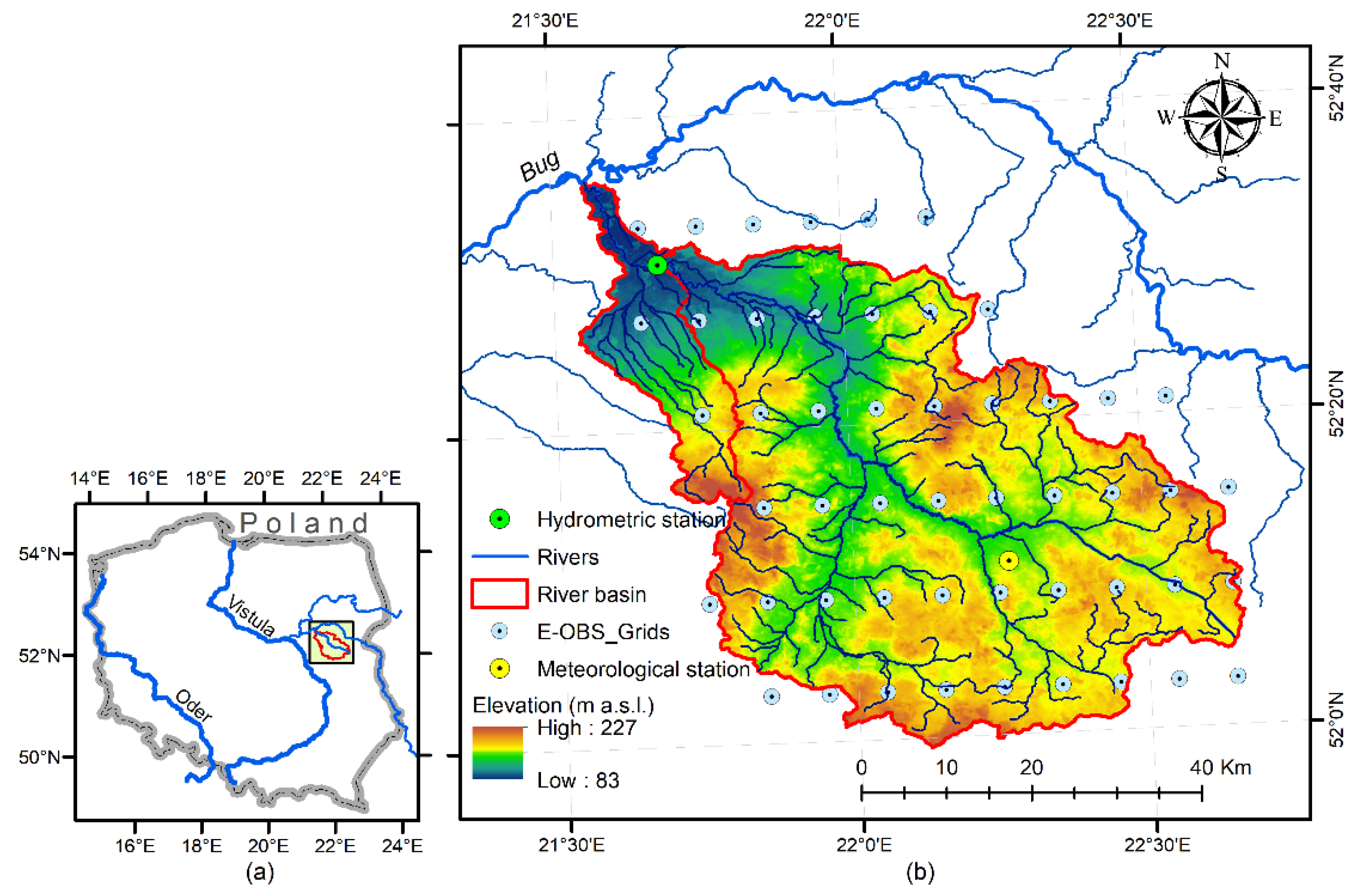This illustration features two detailed maps of Poland side-by-side, presented in a horizontal rectangular layout. On the left, a small overview map provides a general geographical context, highlighting the locations of major rivers such as the Oder and Vistula, and showing coordinates ranging from 14 to 24 degrees east and 50 to 54 degrees north. The map also includes a key detailing elements like latitude and longitude.

The right side showcases a larger, more detailed close-up map that elaborates on Poland's topographic and hydrographic features. This map includes elevation data, represented by varying colors to indicate different heights, with the elevations ranging from 83 to 227 meters. It also maps out rivers, river basins, and hydrometric stations, with specific rivers like the Vistula, Oder, and Bug prominently labeled. The larger map spans coordinates from 21 degrees 30 minutes to 22 degrees 30 minutes east and from 50 degrees 40 minutes to 52 degrees north. Additionally, the map features a north-east-south-west compass, a scale of 40 kilometers, and various symbols denoting meteorologic and hydrometric stations. The color-coded elevation and the presence of a detailed key make it a comprehensive yet complex depiction of the region's geographic features.